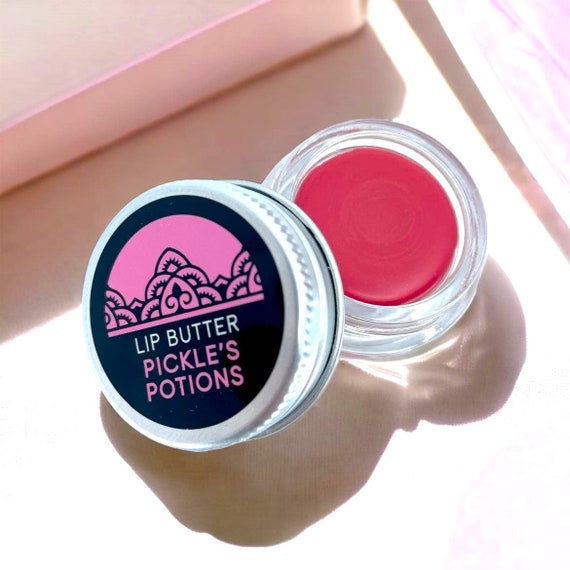The image depicts a small circular glass container of bright red lip butter with a silver lid that has been unscrewed and tilted against the left side of the container. The background is a pinkish color, possibly a table or cloth, with shadows cast by the strong sunlight hitting the setup. The lid features a black label with a pink and black design, and it prominently displays the text "Lip Butter Pickles Potions" in a mix of purple, pink, and light bluish-green. The design on the label includes intricate patterns reminiscent of fleur-de-lis or henna. The untouched lip butter inside the container gleams, indicating its vibrancy and smooth texture. The entire scene is closely cropped, with the shadows from the pot and the lid creating a dynamic composition, enhancing the overall presentation of the lip butter product.